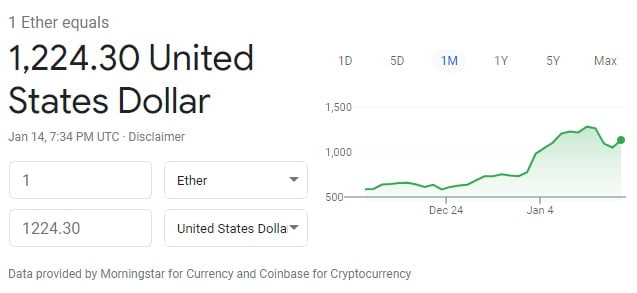The image displays a detailed section of a cryptocurrency web page. At the top, in gray letters, it states "1 Ether equals," followed by "1,224.30 United States Dollar" in bold black text. A gray date stamp reads "January 14th," accompanied by a timestamp of "7:34 p.m. UTC" and a disclaimer note.

Beneath this, there are two horizontal boxes: the first box contains the number "1," while the second box, to the right, includes a drop-down arrow and the word "Ether." Just below is the repeated number "1,224.30," with "United States Dollar" in another drop-down arrow box to the right.

Following these elements is a graph display with various selectable time frames: "1D," "5D," "1M," (currently being displayed), "1Y," "5Y," and "Max." The vertical axis shows numerical values, marked notably at "1,500."

The graph itself features a yellow line charting the value of Ether. Starting at about "550" on "1D," it tracks movements from December 24th to January 4th. Initially steady through the end of December, the line begins to rise in January, experiences a slight dip, and then climbs upward again.

At the bottom of the image, there is a note stating, "Data provided by Morningstar for currency and Coinbase by cryptocurrency."